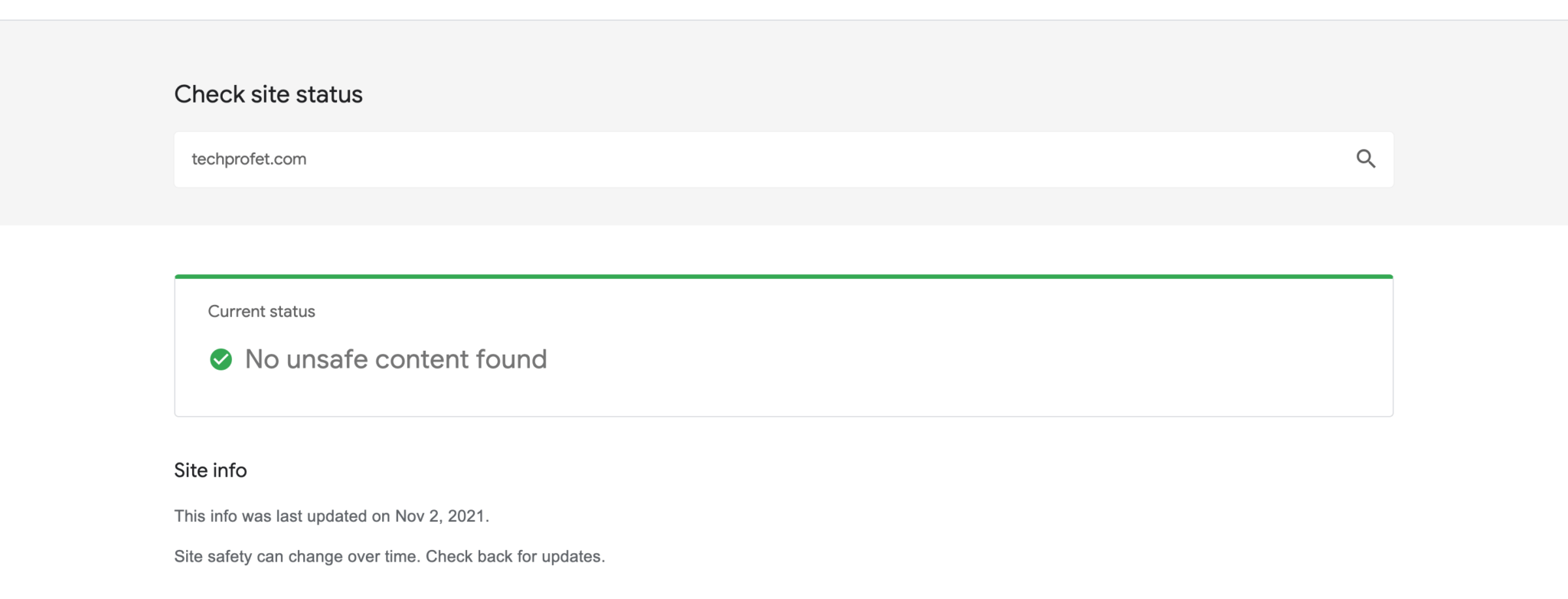The image is a horizontally oriented screenshot with unique dimensions, having an approximate height-to-width ratio of 30:70. At the top, a light gray bar spans horizontally, displaying the text "Check Site Status" in black. Directly beneath this bar, there is an elongated horizontal search bar. On the left side of this bar, the URL "techprofet.com" is displayed, spelled as T-E-C-H-P-R-O-F-E-T dot com, with a search option towards the right.

Below the search bar, the background is white, featuring a small white box with a horizontal green line along its top edge. Inside the box, it says "Current Status" along with a note indicating "No unsafe content found." A green check mark accompanies this text. Beneath the box, in black text, it reads "Site Info." Following this, a message indicates, "This info was last updated November 2nd, 2021. Site safety can change over time. Check back for updates."